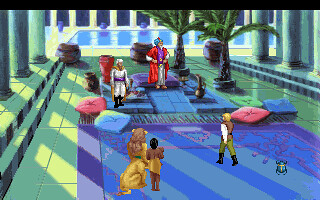In this vibrant still from a cartoon or video game, a richly detailed indoor setting is depicted. In the background, there is a tranquil pool that sets the scene near the rear of the building. Moving toward the foreground, the floor is adorned with green tiles, leading up to a number of ornate black planters that host tall, lush palm trees. 

A prominent platform dominates the middle ground, featuring a regal figure standing authoritatively near a small purple throne or cushion. This individual, presumably a king, commands the attention of the scene. Standing vigilant nearby, dressed in white attire, is another character who appears to be a guard, providing protection for the royal figure.

The scene also includes a man approaching the king’s platform, distinguishable by his white shirt, brown vest, green pants, black boots, and blonde hair. His presence suggests he is either seeking an audience with the king or is part of the court.

In the bottom left corner of the image, there is another intriguing element: a person standing beside a large lion. The lion is notable for its imposing height and is seen sitting tranquilly next to the human companion, adding an air of majesty and intrigue to the overall scene.